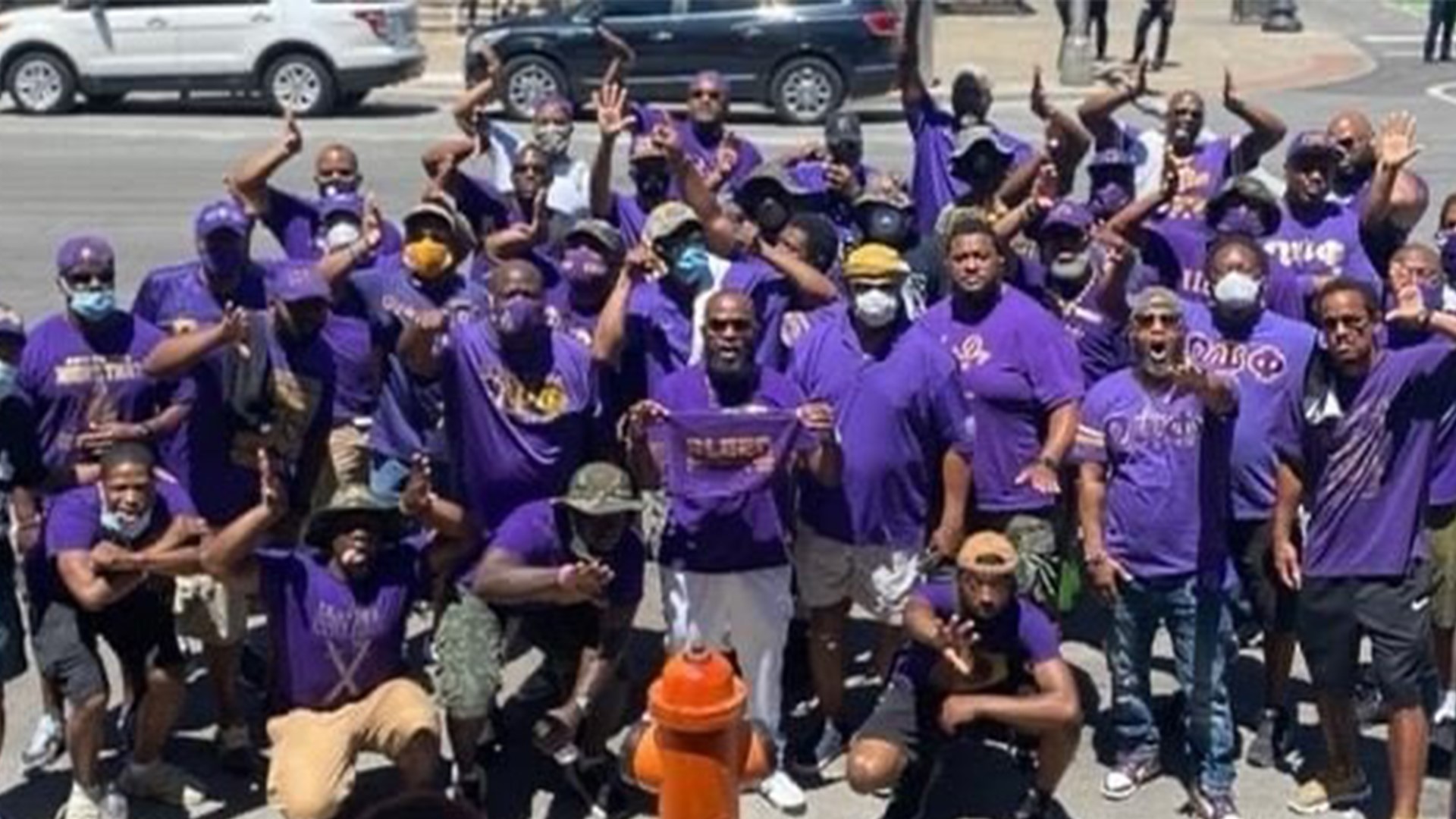The image captures a vibrant street scene featuring a group of African American men all dressed in various styles of purple shirts, some plain and others adorned with different graphics. They are gathered in an intersection, standing and kneeling in front of an orange fire hydrant, all facing the camera. Many of them are wearing masks, reminiscent of the COVID-19 pandemic. The men are predominantly wearing shorts or summertime long pants, suggesting a warm day. Behind them, the sidewalk is bustling with additional people associated with the group. Two parked SUVs, one white and one dark blue with white rims, provide a backdrop. The quality of the image is notably poor and blurry, but the celebratory and possibly activist spirit of the group is clearly conveyed through their raised hands and unifying purple attire.